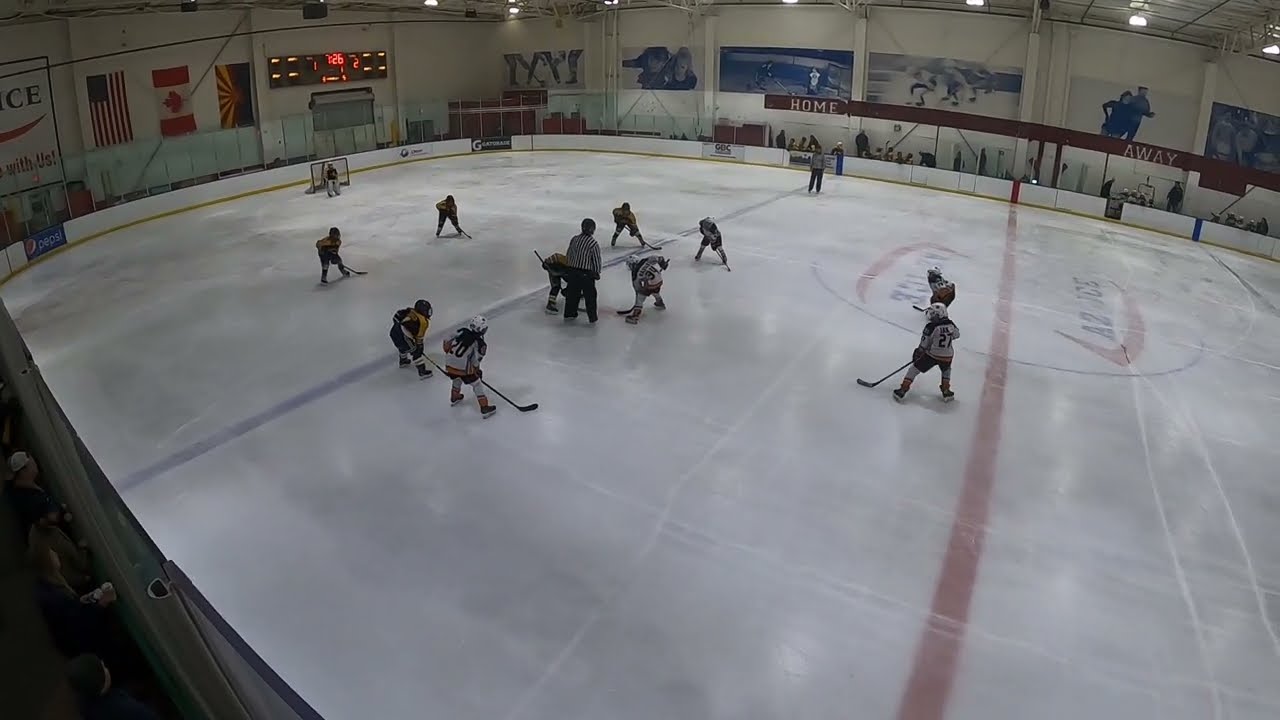The image captures the early moments of an indoor hockey game with numerous players on the ice rink between the "Home" and "Away" zones, as indicated by the signs on the far wall. Taken from a high vantage point in the stands, the scene is brightly lit by overhead lights. At the center, a referee stands between two players, poised for the face-off, both hunched over their hockey sticks and focusing intently on the puck. One team is dressed in white jerseys with dark letters, wielding black sticks, while the opposing team sports tan yellow colors. On the left side, an electronic scoreboard displays the American, Canadian, and Arizona state flags, emphasizing an international or friendly match atmosphere. The rink also features images of hockey players and ice skaters on the walls, suggesting it doubles as a multipurpose ice skating venue.